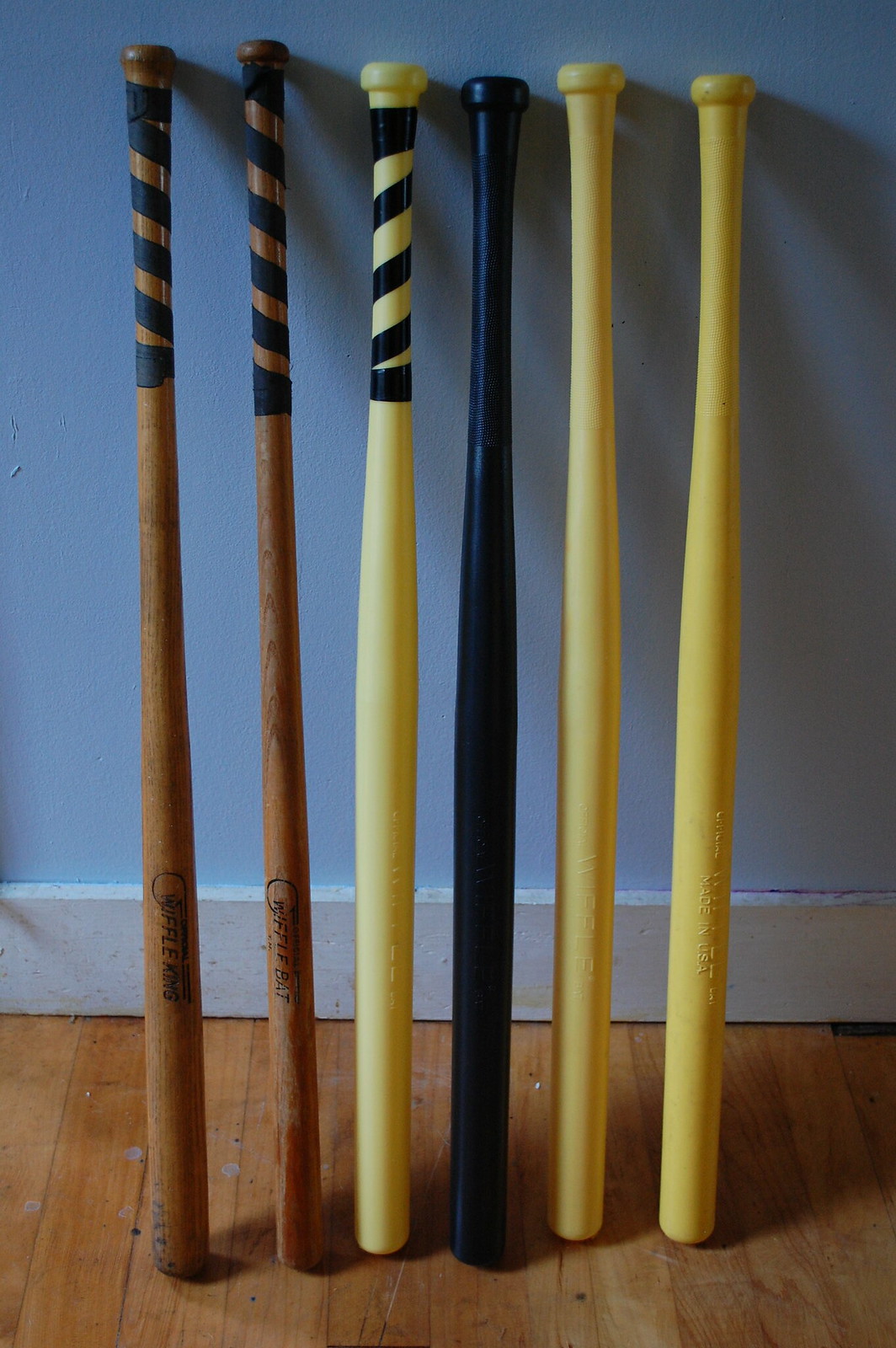This photograph depicts six baseball bats—five wooden and one plastic—leaning vertically against a light blue wall with a white baseboard. They stand on a worn wooden floor. The first two bats on the left are brown wood, each with black tape spiraled around the handle. The third bat is a light cream color, also with a black taped handle. The fourth bat is entirely black. The fifth and sixth bats share a slightly darker cream hue, and they lack any handle wrapping. Notably, the first wooden bat is titled "Wiffle King" and is slightly thicker than the others, while the second is labeled "Wiffle Bat" in black text. The image captures the organized yet varied appearance of these sporting tools against the serene backdrop.